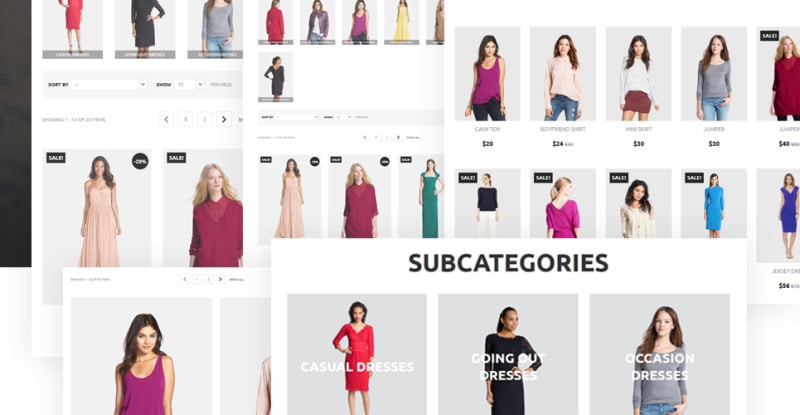This image depicts a women's clothing website showcasing an extensive collection of apparel. The layout is somewhat cluttered, with multiple overlapping screens, suggesting different sections of the site being viewed simultaneously. Notably, there is a specific category highlighted called "Cam Tops" priced at $20, although the display is overlapping with another section titled "Subcategories" that includes Casual Dresses, Going-Out Dresses, and Occasion Dresses. Interestingly, the image associated with Occasion Dresses features a woman in blue jeans and a gray long-sleeve t-shirt, which notably does not align with typical dressy attire. Similarly, the styles represented under Casual Dresses and Going-Out Dresses don't quite match their categories, contributing to a sense of confusion in the site's organization. In total, there are 27 images displayed, each showcasing a variety of women's clothing. The overall presentation appears busy and somewhat disjointed, with a mixture of clothing styles that do not strictly adhere to their respective categories.